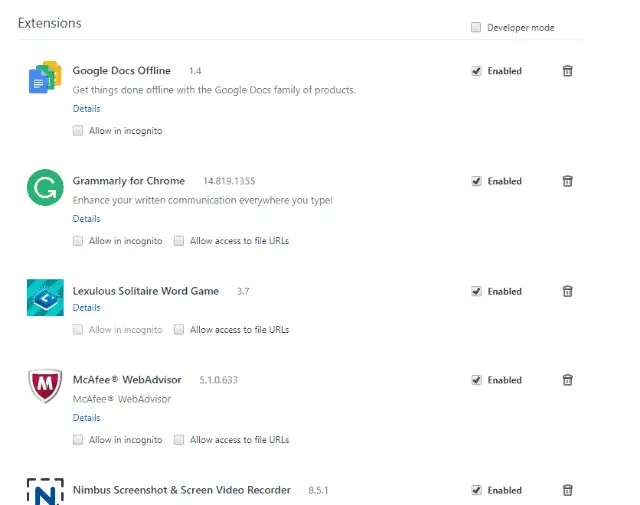Screenshot of a browser extension management page. The background is all white, with black text. At the top left, it says "Extensions". On the top right, there is an unchecked gray checkbox labeled "Developer mode". A thin gray line separates the header from the list of extensions.

The page features five extensions arranged vertically:

1. **Google Docs Offline** 
   - Icon: Google Docs
   - Options: 
     - Checkbox labeled "Enabled"
     - Trash can icon
     - Blue "Details" button
     - Checkbox labeled "Allow in incognito"

2. **Grammarly for Chrome**
   - Icon: Grammarly (green)
   - Options:
     - Checkbox labeled "Enabled"
     - Trash can icon
     - Checkbox labeled "Allow in incognito"
     - Checkbox labeled "Allow access to file URLs"

3. **Lectulus Solitaire Word Game**
   - Icon: Lectulus Solitaire
   - Options:
     - Checkbox labeled "Enabled"
     - Trash can icon
     - Checkbox labeled "Allow in incognito"
     - Checkbox labeled "Allow access to file URLs"

4. **McAfee WebAdvisor**
   - Icon: McAfee WebAdvisor
   - Options:
     - Checkbox labeled "Enabled"
     - Trash can icon
     - Checkbox labeled "Allow in incognito"
     - Checkbox labeled "Allow access to file URLs"

5. **Nimbus Screenshot and Screen Video Recorder**
   - Icon: Nimbus (partially cut off)
   - Options:
     - Checkbox labeled "Enabled"
     - Trash can icon